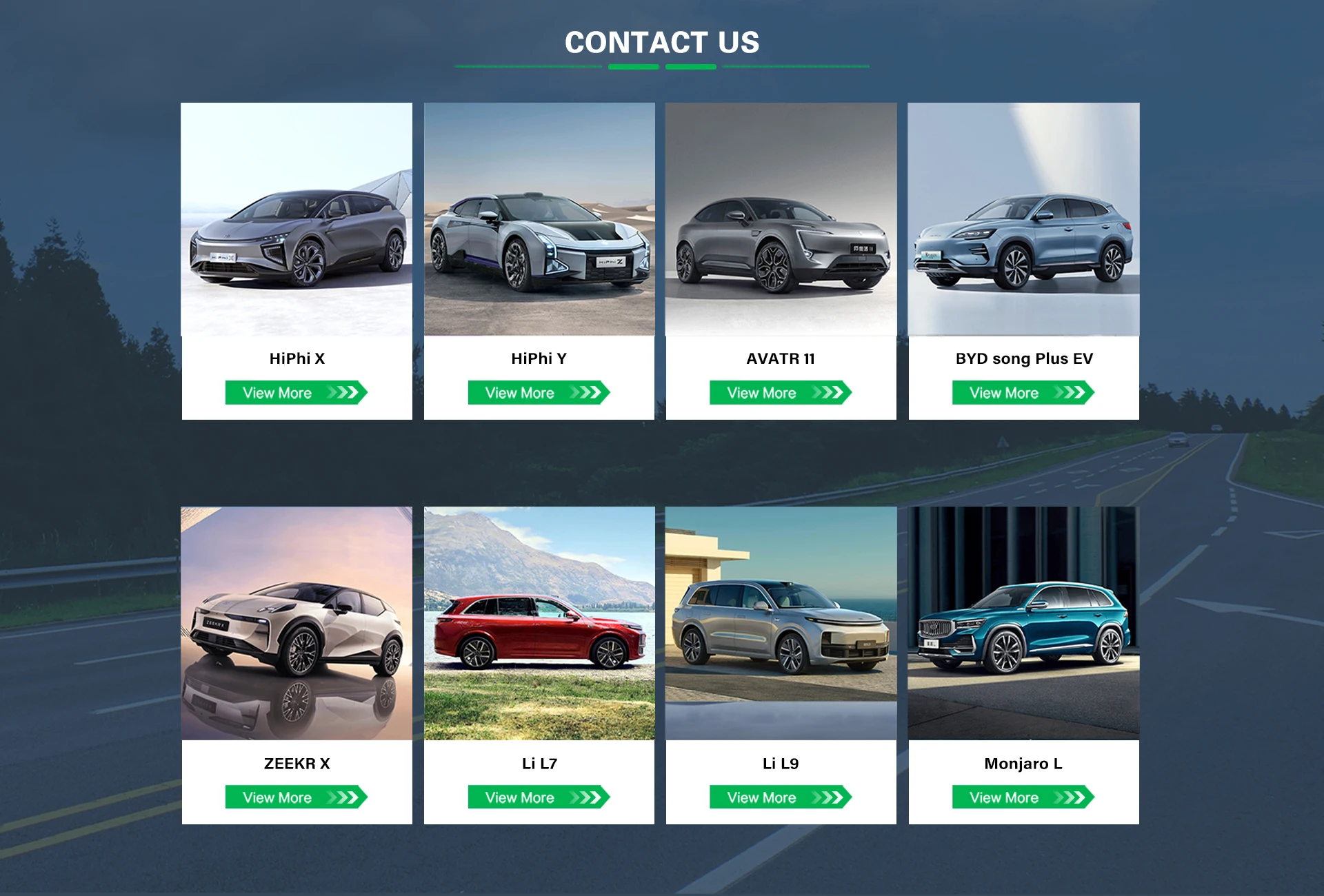The image on this page showcases a lineup of eight distinct cars arranged in two rows and four columns, with four cars on the top row and four on the bottom. The vehicles are:

1. Haifi X
2. Haifi Y
3. Avatar 11
4. BYD Song Plus EV
5. Zeeker X
6. Lai L7
7. Lai L9
8. Manjaro L

These cars are displayed in a variety of colors, predominantly gray and black, with a few blue variations, one red, and one white. A backdrop featuring a semi-transparent photo of a highway scene sets the stage, complete with a blue sky and lush green trees, giving it a serene and picturesque ambiance. 

At the top of the page, the words "Contact Us" are prominently displayed in white font, underscored by a green line. Each car has an associated button labeled "View More," which appears in green and transitions into a right arrow, inviting users to explore further details about each vehicle.